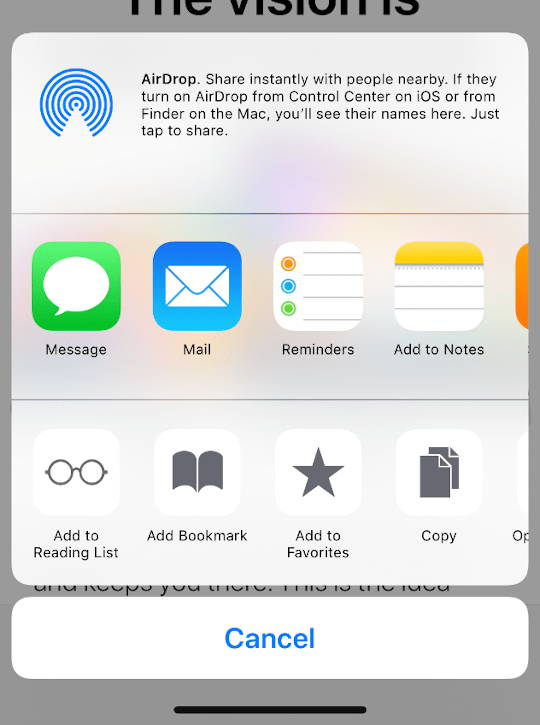The image features a gray background with a white box prominently displayed. This box is divided into various sections, each detailing a different sharing option available on iOS or macOS. Here's a more refined description:

At the top, we see a section labeled "AirDrop" enclosed in a white box. The caption within this section reads: "Share instantly with people nearby. If you turn on AirDrop from Control Center on iOS or from Finder on the Mac, you'll see their names here; just tap to share."

Below this, there is a green box featuring the "Message" option, represented by a chat icon. Adjacent to it, a blue box contains the "Mail" option, symbolized by an envelope icon.

Continuing down, another white box with a set of lines and a yellow header indicates the "Reminders" feature. Additionally, there is a section titled "Add to Notes," also within a white box. 

Moving further, we encounter a white box displaying glasses, which corresponds to the "Add to Reading List" option. Next to this is another white box with a book icon labeled "Add Bookmark." Following that, a white box with a star icon is marked "Add to Favorites."

Further options include a white box featuring two gray pieces of paper, labeled "Copy." At the bottom of the box, a white rectangle contains the word "Cancel" in blue, placed centrally. A black bar at the bottom middle of the box completes the layout.